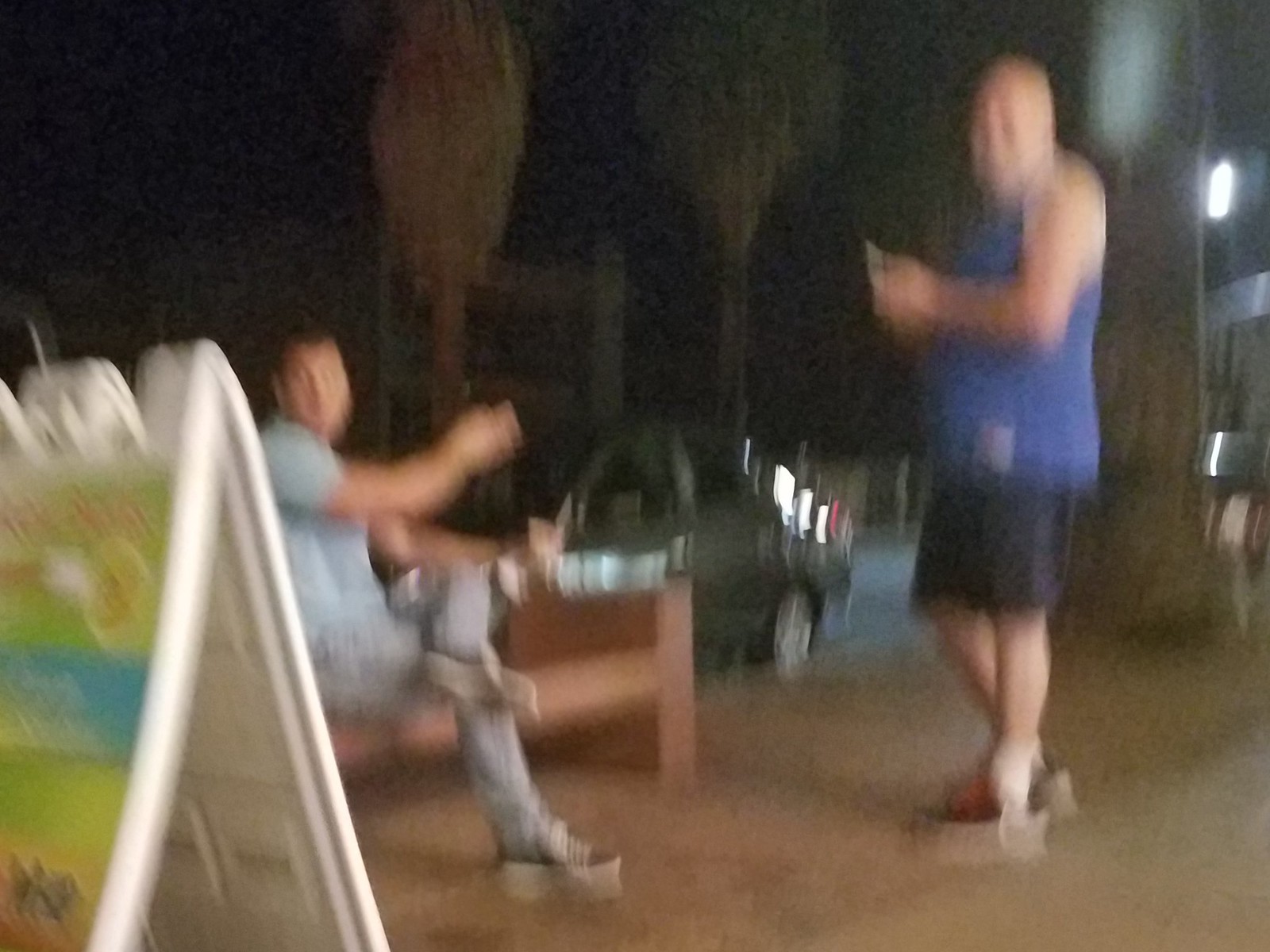In this somewhat blurry photograph, we observe two individuals in a casual outdoor setting. On the left-hand side, a person is seated on a brown bench. This individual is wearing a gray T-shirt and has their right leg crossed over their left knee, donning black shoes. Positioned on the right, another person stands, dressed in a blue tank top and black shorts, complemented by red and black shoes with white socks.

At the bottom left corner of the image, there is a white sign featuring several colored labels—difficult to decipher but arranged with green and orange at the bottom, followed by blue, and another green label at the top. The ground beneath them appears as a uniform brown color. 

Behind the two individuals, a dark gray car is partially visible. Additionally, a tree starts to come into view on the right-hand side of the image, while a few more trees are discernible in the distance. A tall, wooden sign or part of a structure is faintly visible, set against a dark, almost black backdrop that suggests the approaching night or heavily shaded area.